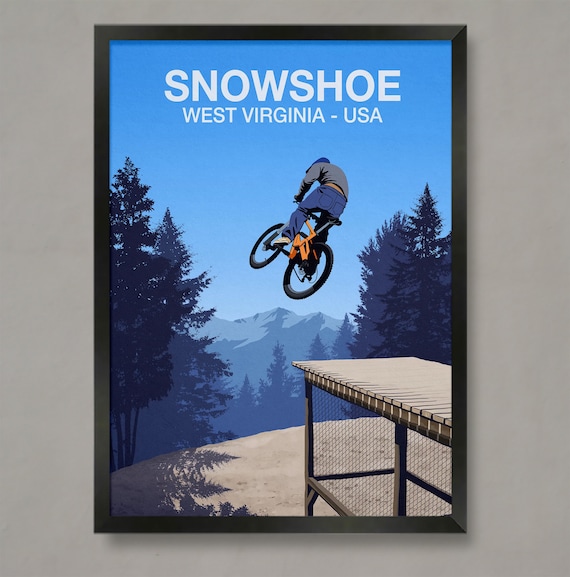This framed poster, set against a grey wall, showcases an illustration titled "Snowshoe, West Virginia, USA." The thin black frame draws the viewer into a dynamic scene: a figure on an orange BMX bike, mid-jump after launching off a constructed ramp on a snowy mountain. The rider, depicted with their back facing us, wears blue trousers, a grey top, and a blue helmet, capturing the thrill of the moment as they soar through the air. Below them stretches a sandy-colored path, and in the background, blue skies, snow-capped mountains, and alpine trees frame the scene, grounding the exhilarating leap in a picturesque, wintry landscape. The predominant colors of the poster are blue, orange, and beige, creating a vibrant, yet harmonious composition that captures the adventurous spirit of Snowshoe.